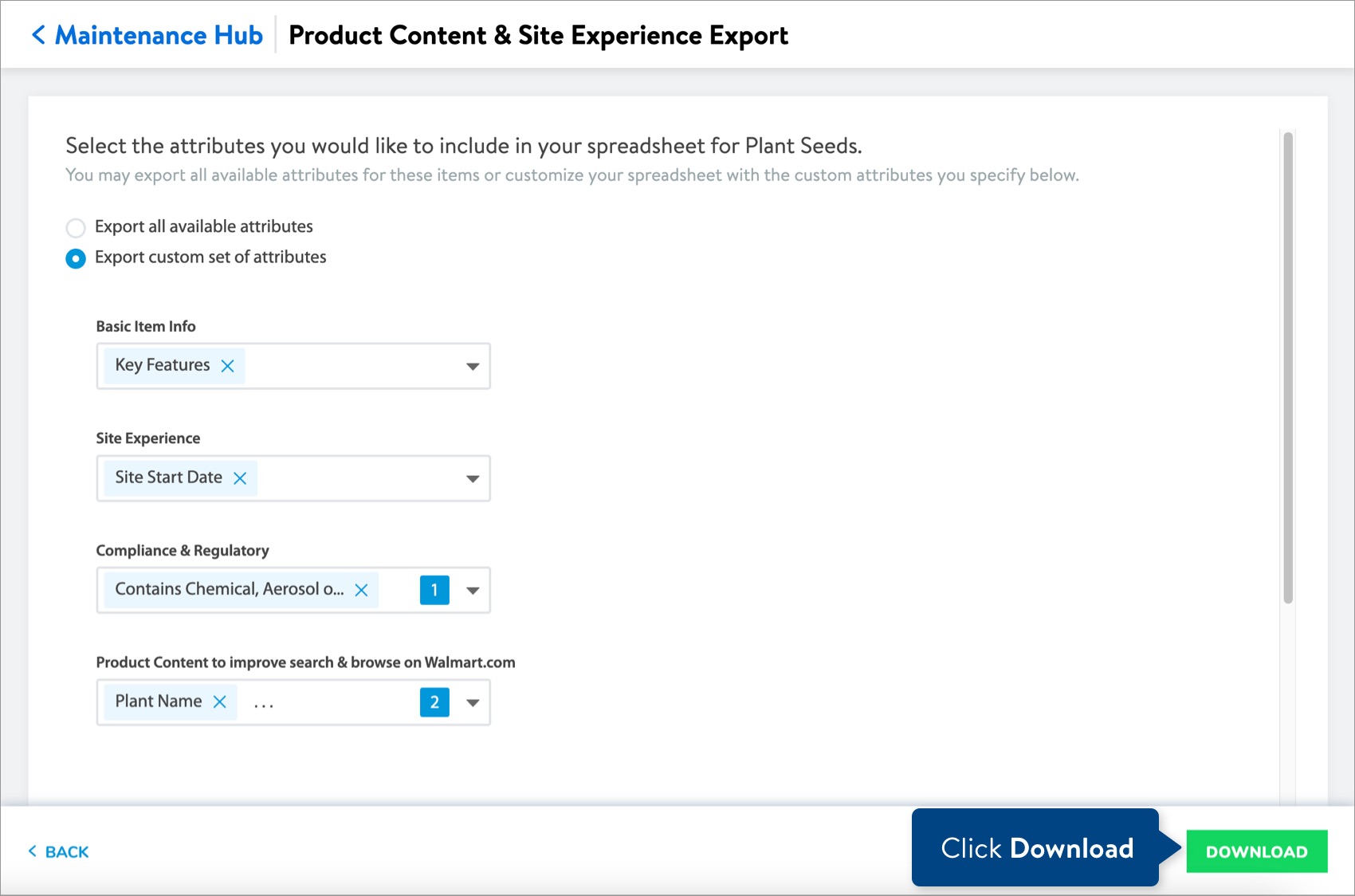**Screenshot Description:** 

The image is a screenshot of a webpage from the "Maintenance Hub" section of a website. This particular section is titled "Product Content and Site Experience Export." The page provides options to select specific attributes for inclusion in an export spreadsheet related to a product referred to as "Plant Seeds." Users are given the option to either export all available attributes or create a custom export set of attributes. 

In this case, the "Export Custom Set" option is selected. The interface allows users to input basic item information, including "Key Features," "Site Experience," "Site Start Date," and "Compliance and Regulatory" details, which cover aspects like "Chemicals and Aerosol." It also addresses "Product Content to Improve Site and Browse on Walmart.com," specifically including the "plant name."

Towards the bottom of the page, after selecting the desired custom attributes, there is a prominent, white-button set against a blue background labeled "Click Download," accompanied by a green arrow icon indicating the download action. These functionalities provide clear instructions for customizing and exporting a set of attributes into a spreadsheet related to "Plant Seeds" for Walmart.com.